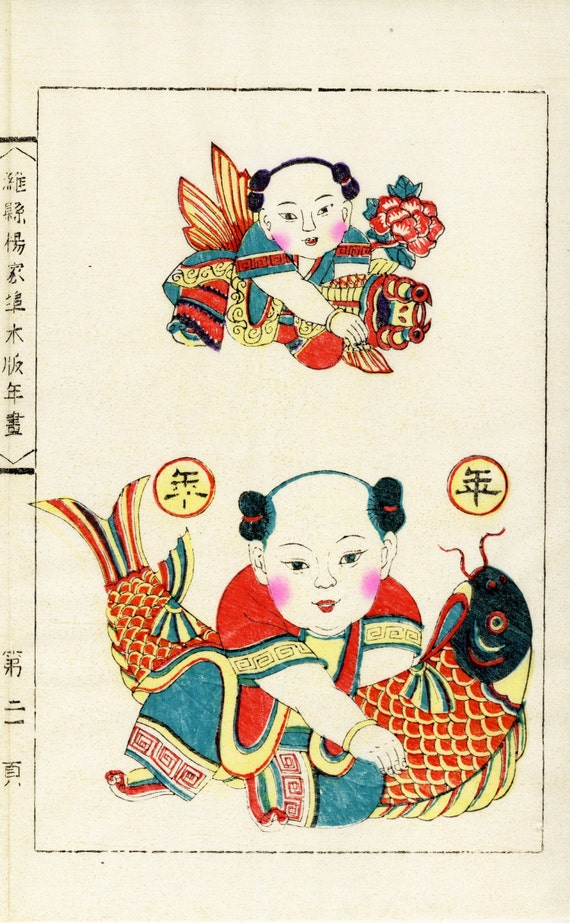The illustration depicts two detailed scenes on a single page, reminiscent of traditional Chinese or Japanese artwork. The artwork is encased within a thin black rectangular border set against a light tannish-yellow background. Vertical columns of Asian script adorn the left side and bottom left corner of the image.

At the top of the illustration, a smaller figure, possibly male or female, is depicted with black hair styled into two tied buns on either side of the head, fastened with red ribbons. The figure has a white face adorned with rosy magenta cheeks and red painted lips, wearing an aquamarine shirt and red pants. The upper figure is holding a smaller fish, with the fish's tail extending behind the figure. A red lotus flower is situated in the upper corner of this scene.

The lower half of the scroll features a larger figure resembling a bald child with small bun-like hair tufts on the sides of the head, characterized by purple blush on the cheeks and red lips. This figure's attire includes a red shirt and aqua-colored pants, decorated with swirling patterns. The figure appears to be wrestling with a large, vibrant red catfish displaying a black face and golden scales. The fish is wrapped around the child's body, extending from the right side under the arm to the left side. Additional colorful elements such as flowers, possibly a basket, and intricate designs enhance the vivid imagery in both scenes. The overall aesthetic of the illustration indicates it may be an older piece, rendered in a colorful ink style, conveying a storytelling element deeply rooted in Asian cultural art.